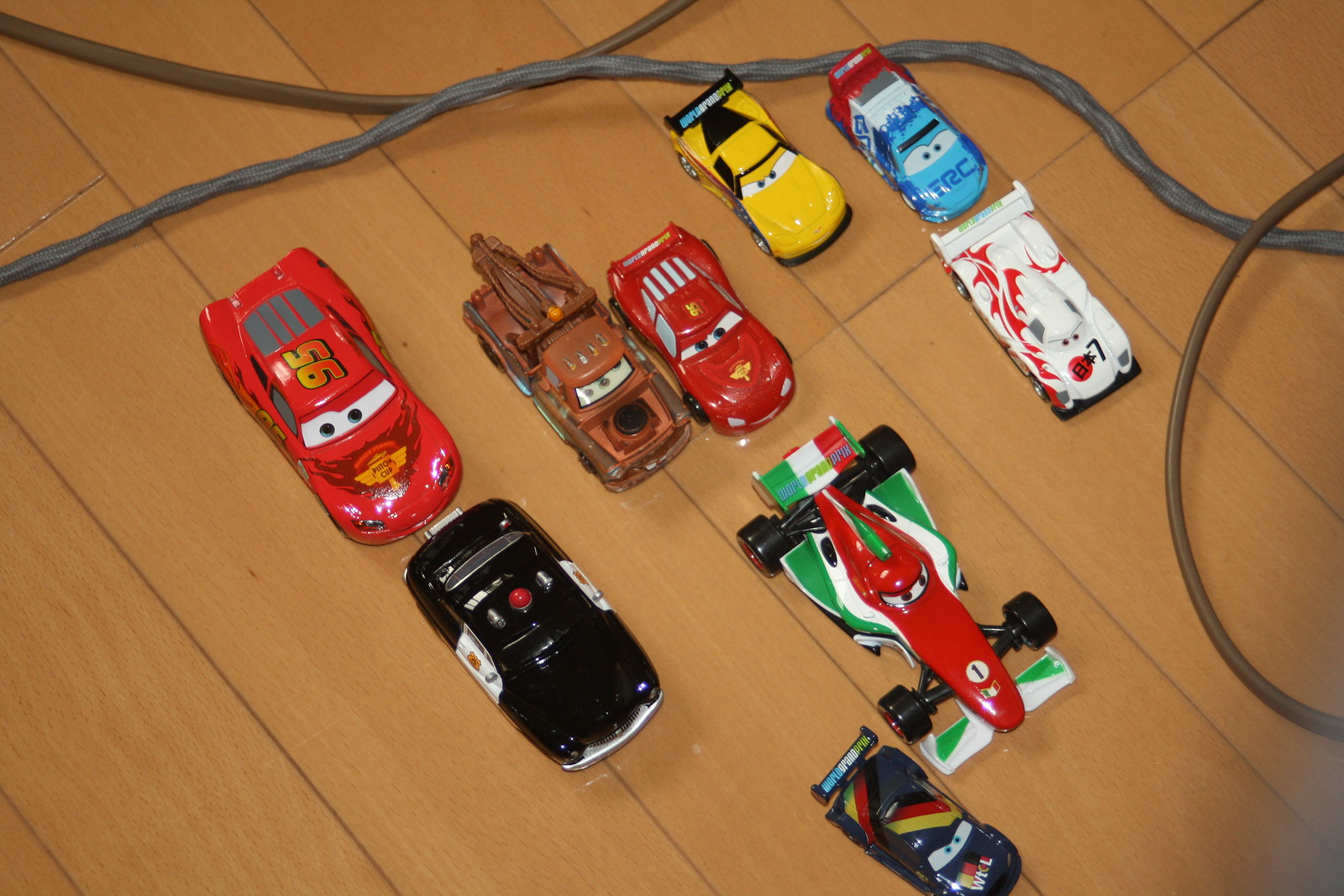The image is a close-up, brightly lit, amateur photograph capturing nine toy cars inspired by the movie "Cars," arranged haphazardly on a wooden panel floor. Each car features distinct, characterful eyes on their windshields. The assortment includes a prominent red car with the number 95 on its top, a brown tow truck, a yellow and blue race car, and a distinct black car. Additionally, there's a green and red racecar, a lightweight white race car, and a smaller gray race car. Also visible are a cop car on the left side and a grayish Indy-style car. Two electrical cables snake above the toys, hinting at a casual, lived-in environment. The cars are positioned at a 45-degree angle, facing the bottom right, laid out in two uneven rows, adding a touch of playful disarray to the scene.